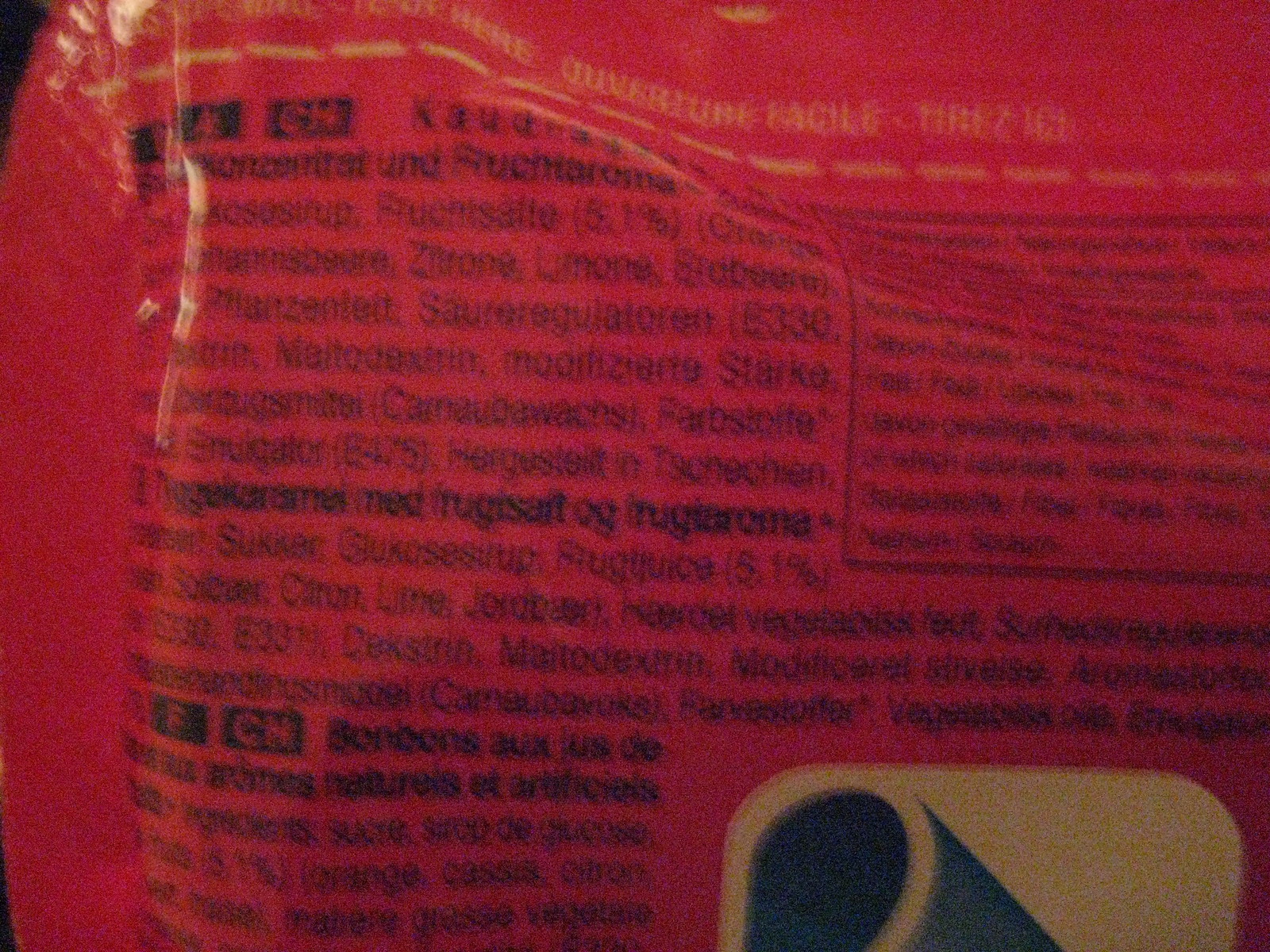This is an extremely blurry image depicting the back of a red, crinkly plastic bag, presumably for a consumable product. The text, which appears to be an ingredients list written in German or a Germanic language, is black and hard to decipher due to a doubled, double-vision-like effect. A yellow dashed line is visible at the top, accompanied by some yellow text. In the top right quadrant, there's a small black box containing additional text. In the bottom right corner, part of a design can be seen, featuring the top of a yellowish square with rounded corners. Additionally, there's a black opening on the left side near a curved triangle-like shape. The top left corner of the image includes a portion of a black background.